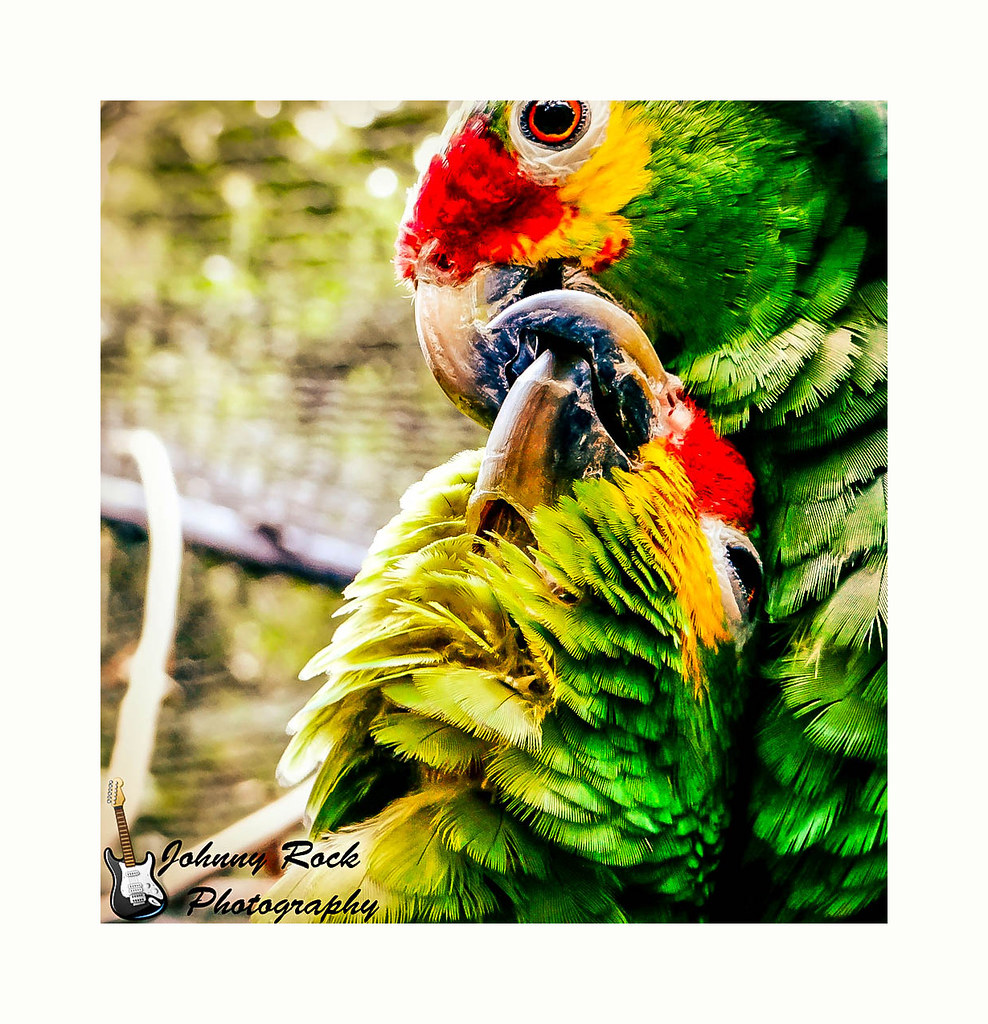The close-up image vividly captures two medium-sized parrots engaged in grooming, evoking an intimate and tender moment as if they are kissing. The birds are predominantly bright green with striking red feathers above their beaks and yellow feathers just beneath their eyes. One parrot, positioned towards the center, looks downward while the other, to the right, cranes its neck upward. Their vibrant plumage appears almost oversaturated, making each feather stand out with vivid intensity. In the background, a blurry mix of greenery and the faint outline of a metal cage can be discerned, adding context to their environment. The image's bottom right corner features the text "Johnny Rock Photography" accompanied by a small, illustrative guitar icon. This composition ensures that the parrots remain the focal point, with their closely nestled heads and vivid, colorful feathers capturing the viewer's attention.